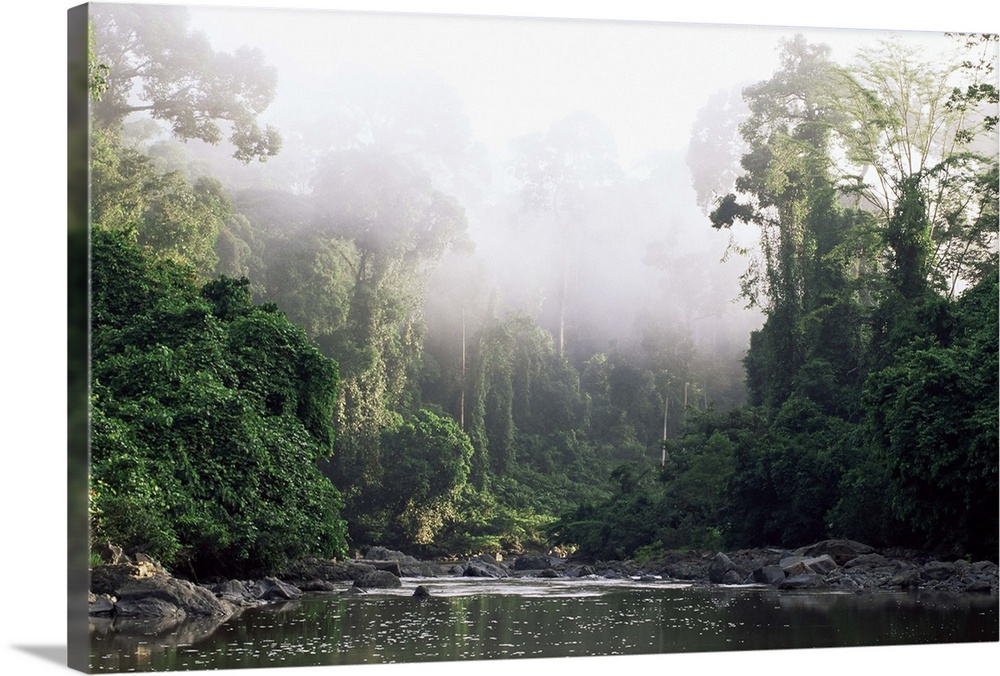The image depicts a highly realistic painting on a large canvas, approximately two inches deep around the edges, that almost looks like a photograph. It showcases a dense, lush, tropical rainforest brimming with greenery. Dominating the center is a body of water, which could be a stream, pond, or lake, with darkish black, still, and reflective surface. The water is bordered by substantial rocks and boulders, with signs of rapids where it meets the rocks. Surrounding the water, tall, verdant trees mix with pine trees, filling the scene with vibrant foliage indicative of spring or summer.

The right side of the image features lofty trees with dense, high brush and some rocky and log-filled debris. On the left, plentiful bushes, trees, and logs transition into the water. The background displays a misty, fog-shrouded horizon with a mist-covered, cloudy sky, and well-lit trees further in the distance, suggesting daylight, possibly at daybreak. The overall effect is one of serene yet dynamic natural beauty, meticulously detailed to evoke the realism of a photograph.